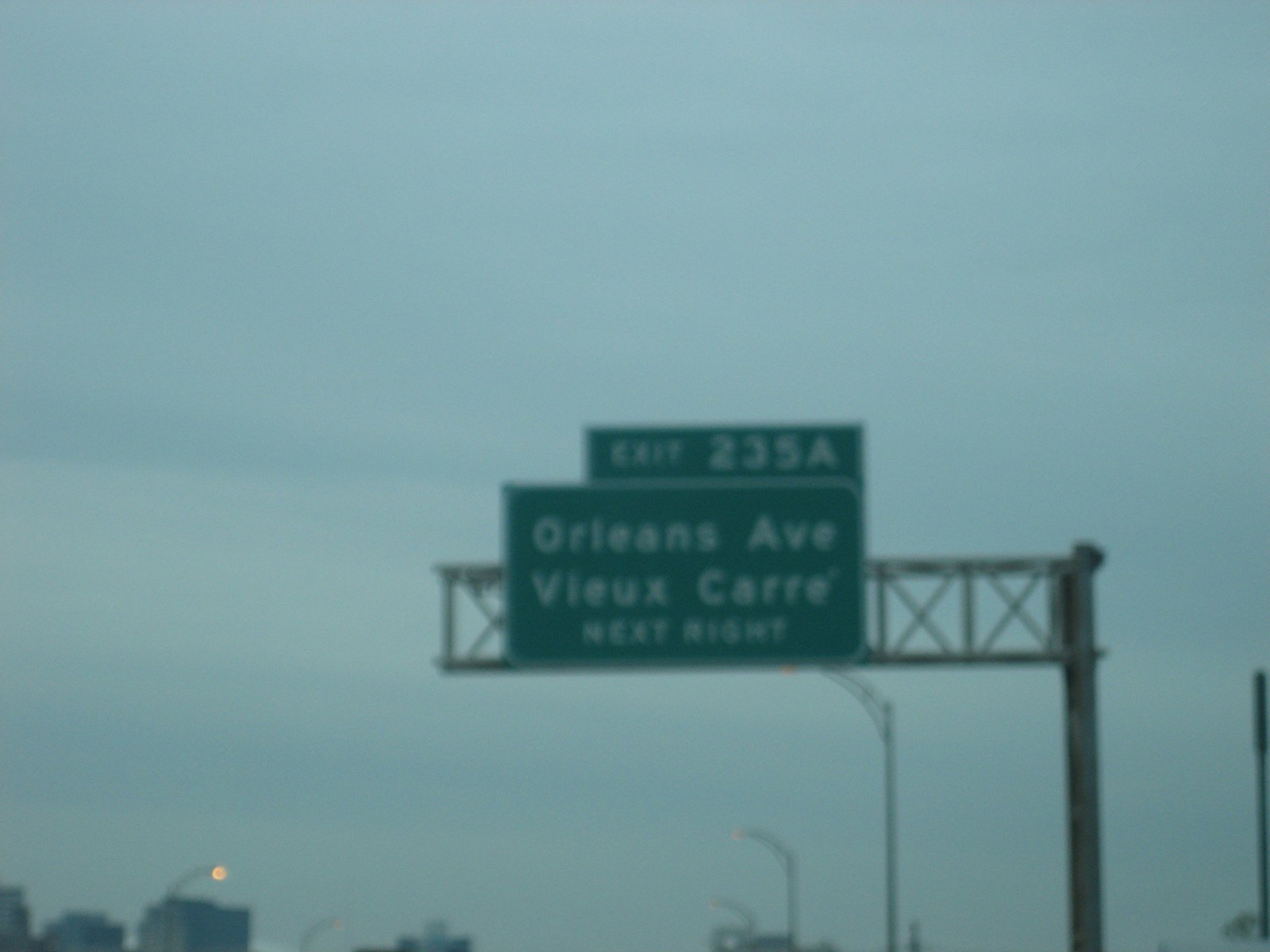In this image, we witness a vivid snapshot of urban infrastructure under a serene sky. Dominating the composition is a prominent green freeway sign displaying directions to "Orleans Avenue," "Le Café," and "Let's be French," with an indication of the next right exit, marked as "Exit 255A." The sign is poised against a backdrop of an expansive sky, adding depth and a sense of openness to the scene. 

Below the freeway sign, the city's architectural landscape emerges with an array of skyscrapers and buildings, adding to the metropolitan atmosphere. Scattered among these towering structures are various metal streetlamps and additional overpass signs, contributing to the complexity of the urban setting. A single streetlamp stands out, casting a warm glow and signifying its activation amidst the encroaching dusk or early evening.

Overall, the image captures the juxtaposition of natural and man-made elements, emphasizing the harmony and tension within a bustling cityscape.